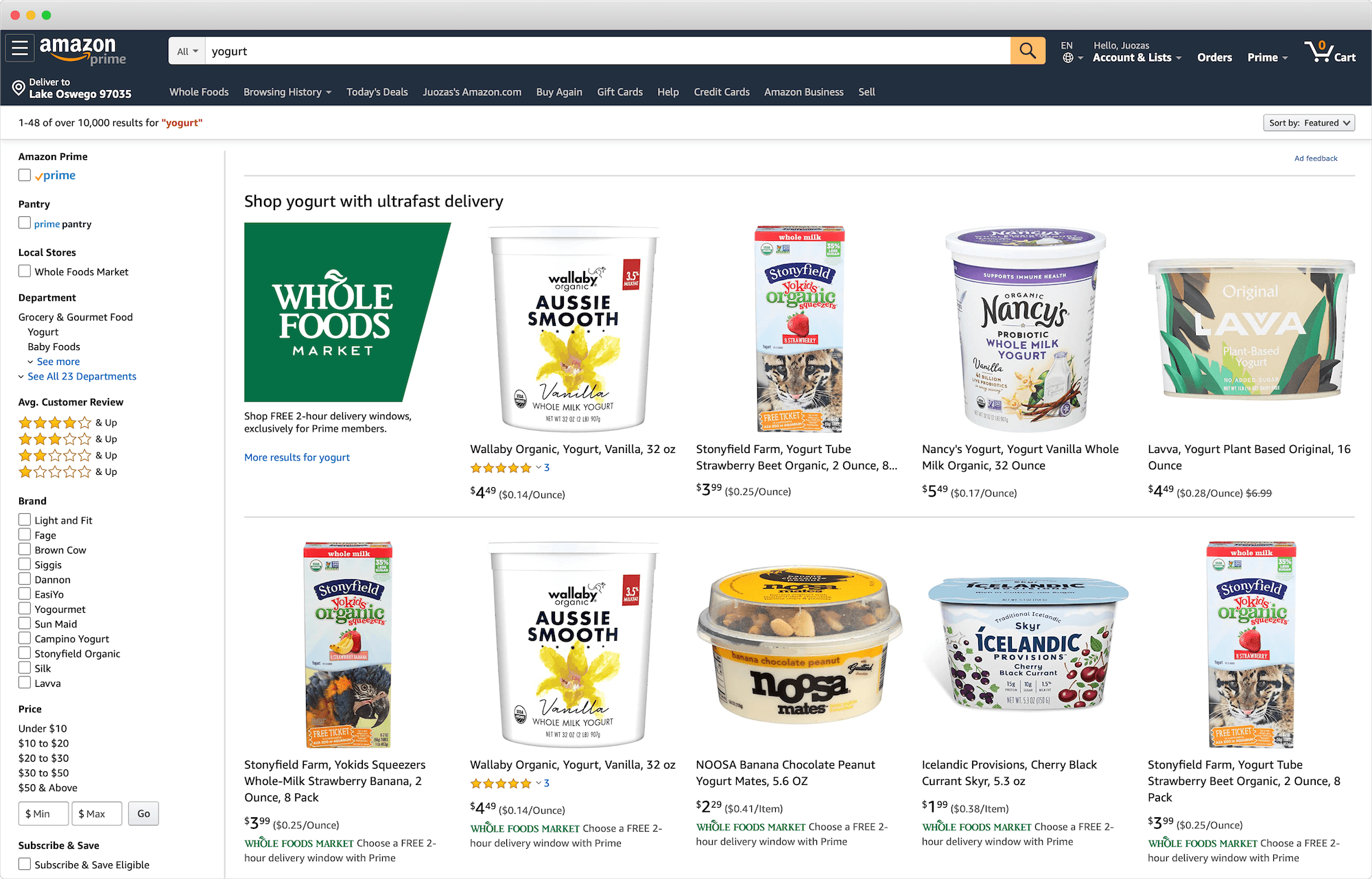Screenshot of a product search on the Whole Foods Market section of the Amazon platform. At the top, the Amazon Prime logo is prominently displayed, indicating that the services are integrated for Prime members. Below the logo is a search bar with the term "yogurt" already entered. The standard Amazon navigation buttons are present: "Account & Lists," "Orders," "Prime," and a shopping cart icon showing zero items in the cart. On the left-hand side, additional filter options are available to refine the search results. The main content area displays nine different yogurt products, each with its own image. Brands visible in the screenshot include Aussie Smooth, Nancy's, Lava, Nopsa, and Icelandic, among others. The Whole Foods Market logo is also visible, signifying the retailer's presence on the platform.